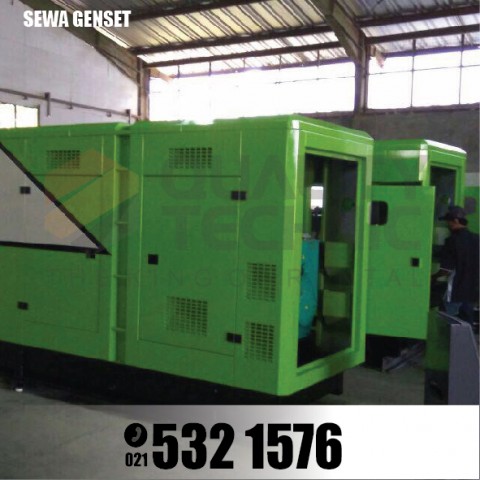The photograph showcases two identical industrial generators situated in what appears to be a warehouse or factory setting. Both generators are rectangular, bright green, and feature large doors at the front, which are currently off. Striking elements on the generators include a large white rectangle on the side with a black border and multiple air vents for heat release. The background reveals high ceilings and walls with windows allowing natural light to flood in. There is a person in dark clothing interacting with the generator in the background. Over the entire image, a watermark reads "QUALITY TECH." Text is overlaid in the top left corner with the label "SEWAGENSET" in white letters, and at the bottom, a semi-transparent white rectangular banner displays the contact number 021-532-1576 in black. The scene conveys a typical industrial environment with essential machinery and operational elements visibly detailed.